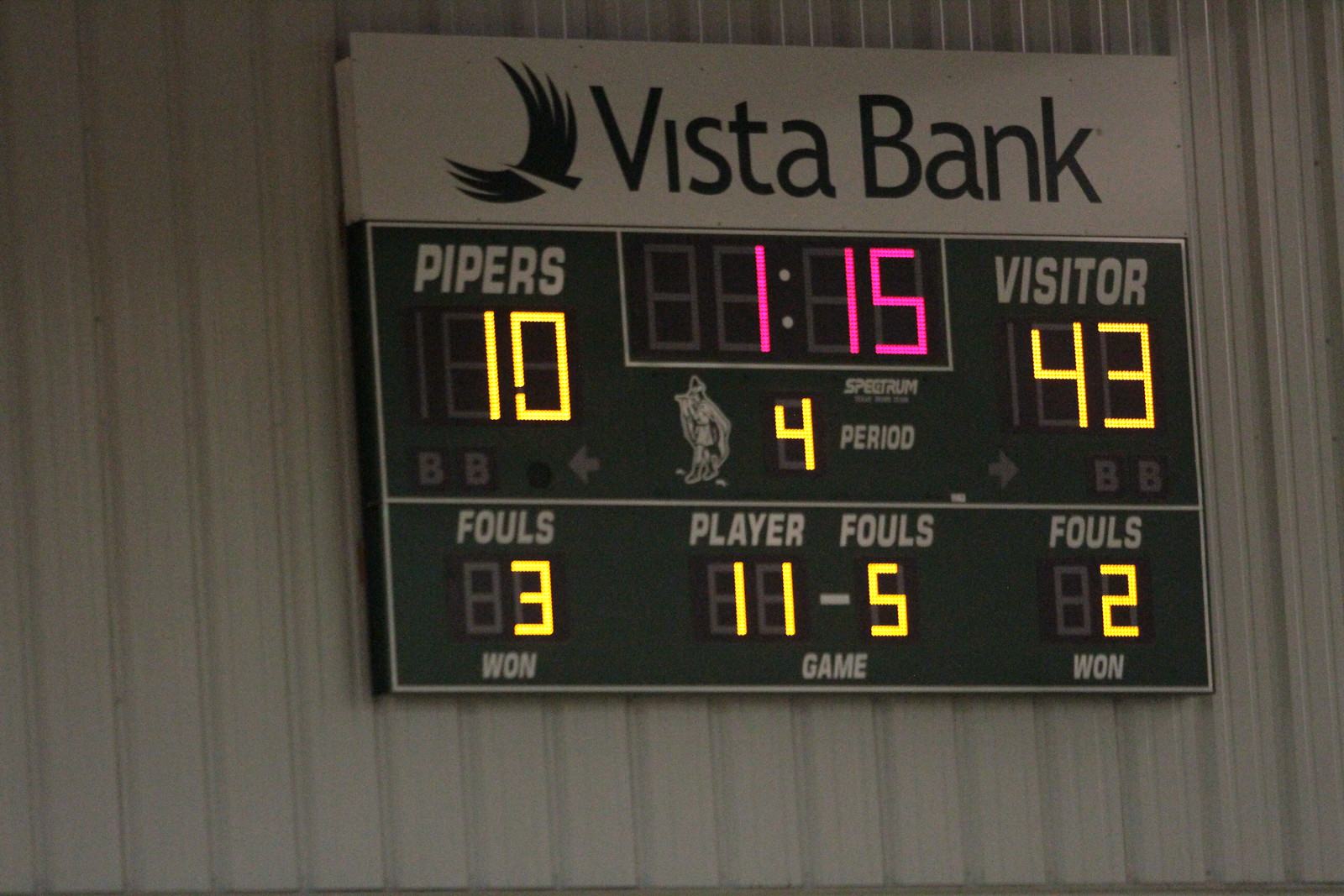In the image, a rectangular scoreboard is displayed against a corrugated white metal wall. A shadow extends from the top left to the top right of the image. The top quarter of the scoreboard features a white background with a graphic of a bird flying left and, to its right, the text "Vista Bank" in black, indicating the sponsor. Below this, the main area of the scoreboard has a black background.

All numerical values on the scoreboard are illuminated in a gold-yellow color, except for the time, which is displayed in pink in the middle top section. On the left side, the team name "Pipers" is displayed in white text, while "Visitor" is shown on the right. The Pipers have a score of 10, whereas the Visitors lead with a score of 43.

The scoreboard indicates it is the 4th period, referred to here as a period though it means quarter. The fouls for the left side show a value of 3, while the right side shows 2. In the middle section, labeled "Player Fouls," the numbers 11 and 5 are displayed. The combination of the black background and the bright display colors makes all the information clear and easy to read.